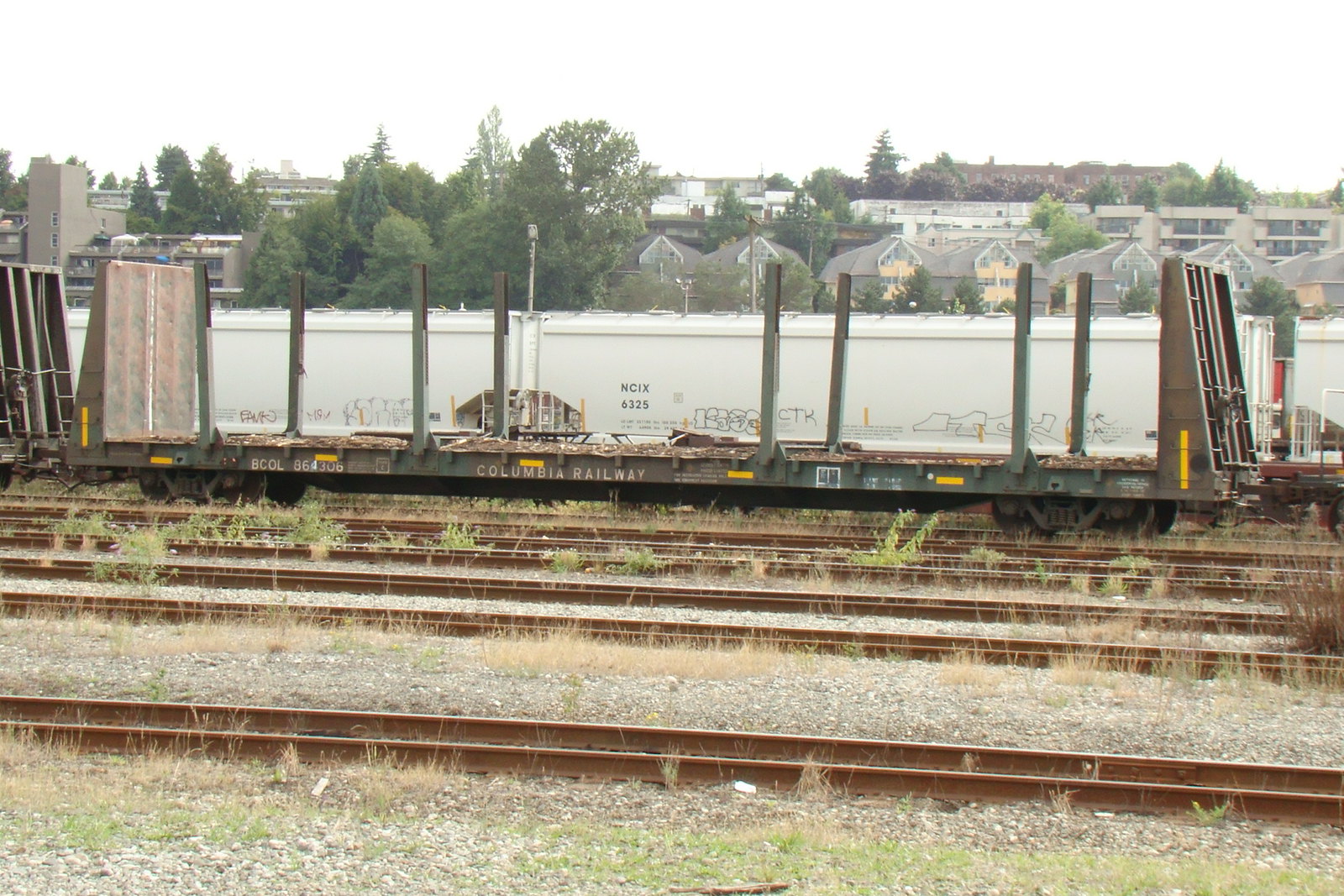The image depicts a train depot featuring several parallel train tracks. In the foreground, the tracks are surrounded by gravel and dirt, with tufts of weeds and grass sprouting intermittently. Dominating the scene is a white train, which bears some black graffiti near the bottom of its cars, although the specific markings are indiscernible. Another train car, seemingly unclosed and barren, is positioned in front of this train, revealing its wheels and a few metal posts in the center. Behind the trains, a residential area with scattered trees and various buildings stretches into the distance. The overall cityscape is dotted with more trees and buildings, culminating at the horizon under a pale, almost white sky devoid of distinct details.